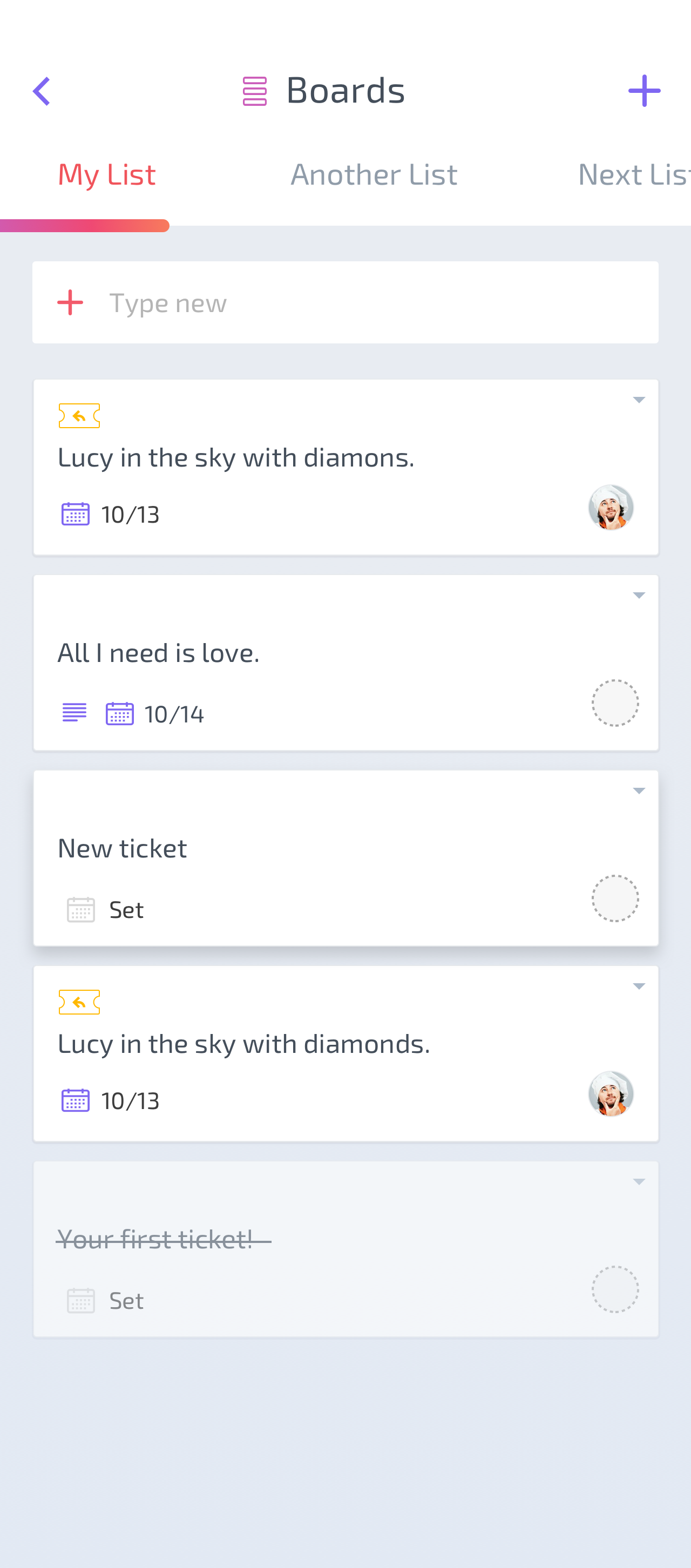This screenshot features a task management application user interface. At the top-left, there is a pink hamburger menu icon. To the right is a blue plus sign, and to the far left is a left-arrow icon. The interface displays several lists, including "My List," which is selected and highlighted in red, while other list names such as "Another List" appear in gray. Notably, the word "lists" is partially cut off, missing the "t."

Under these lists, there’s a prompt to "Type New" with a pink plus sign next to it. The screen lists tasks, such as "Lucy in the Sky with Diamonds" with a completion status shown as "10/13." This task appears next to a user's profile picture. Another task, "All I Need Is Love," is documented as "10/14" and is associated with a gray circle placeholder instead of a profile picture. 

Additionally, there's a section titled "New Ticket Set," following the same format with a gray circle placeholder, and another entry for "Lucy in the Sky with Diamonds" marked "10/13" next to a profile picture. This layout succinctly shows various tasks and their statuses alongside user identifiers, providing a visually organized view of to-do lists and activities.